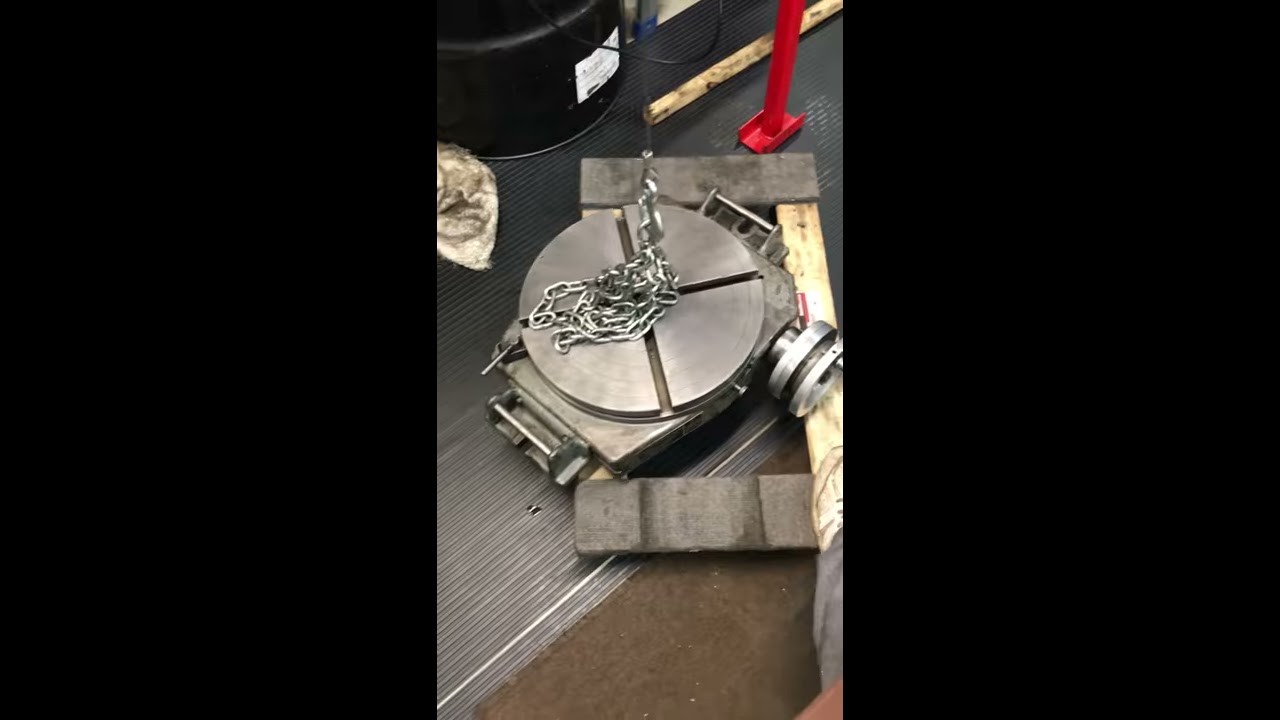The image features a close-up view of a mechanical setup situated in what appears to be a garage or warehouse setting. Central to the scene is a prominent circular metal disc, segmented into four equal parts. Draped over this disc is a silver chain, the end of which leads off the top of the frame, suggesting attachment to another object. The metal disc is mounted on a somewhat rusty base, contrasting with the shinier sections above. Flanking the primary object are various tools and materials including a red metal pipe, a black brick, and wood beams, all scattered across a black or dark gray rubber mat with vertical ridges that enhance its textured appearance. Additionally, a small wheel is visible protruding from the side of the disc, and the entire assembly rests atop a wooden dolly, hinting at the object's considerable weight and the need for mobility. The surrounding area is cluttered, indicating an ongoing project or construction effort, possibly aimed at building or repairing a machine or electronic device.